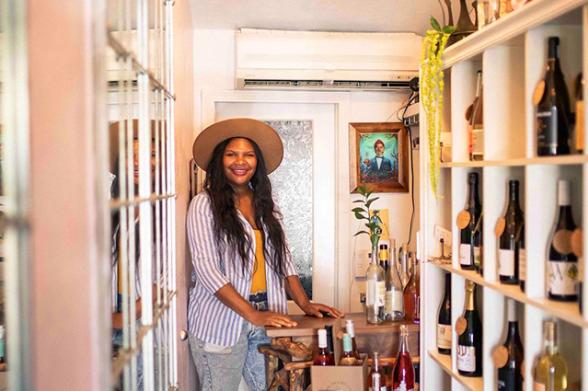The image captures a woman standing in a narrow, cramped space that appears to be a wine shop. She is positioned at the end of a skinny path flanked by shelves holding bottles of wine, each adorned with a small tag or lanyard. On her left, there is an open glass door leading into the space. The woman has darker skin, long black hair reaching almost to her belly button, and she is wearing a wide-brimmed brownish-tan hat. Her outfit includes a blue and white vertically striped pullover shirt layered over a yellow, low-cut tank top, paired with light blue, acid-wash jeans, held up by a belt.

The backdrop features an air conditioning unit mounted high on the wall above a glass-paneled doorway, accompanied by a framed portrait of a man wearing a hat. Directly in front of the woman is a wooden table cluttered with both empty and sealed bottles of wine, and some cardboard boxes are stacked nearby. She smiles directly at the camera, with her hands resting casually on the table, creating a friendly and inviting atmosphere amidst the compact setting.